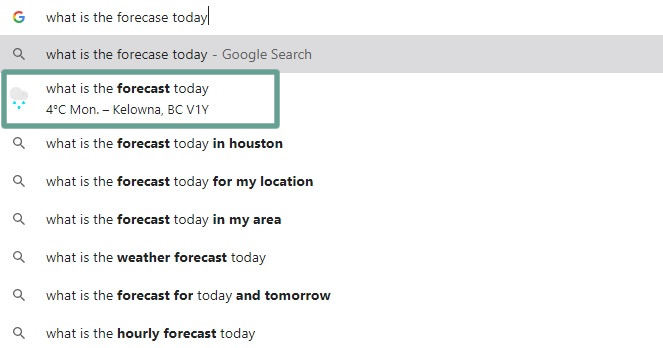An image captures a Google search interface on a white background. The search bar, prominently located in the center of the screen, displays the query "What is the forecast today." To the left of the bar, the iconic multicolored Google logo is visible, partially red, yellow, green, and blue.

Directly below the search bar, a list of autocomplete suggestions is visible in a left-justified column:
1. A gray suggestion that reads "what is the forecast today - Google Search."
2. A highlighted suggestion with a green outline that reads, "What is the forecast today 4 degrees Celsius Monday." Adjacent to this suggestion, a white cloud icon with three blue raindrops signifies rainy weather.
3. "What's the forecast today in Houston."
4. "What's the forecast today for my location."
5. "What's the forecast today in my area."
6. "What's the forecast today."
7. "What's the forecast for today and tomorrow."
8. "What's the hourly forecast for today."

Each suggestion, except the highlighted one with the cloud icon, is preceded by a small magnifying glass icon. The suggestions are displayed in black text, primarily gray, on a clean white background. The image showcases a typical minimalist Google search page, emphasizing the search options related to weather forecasts.